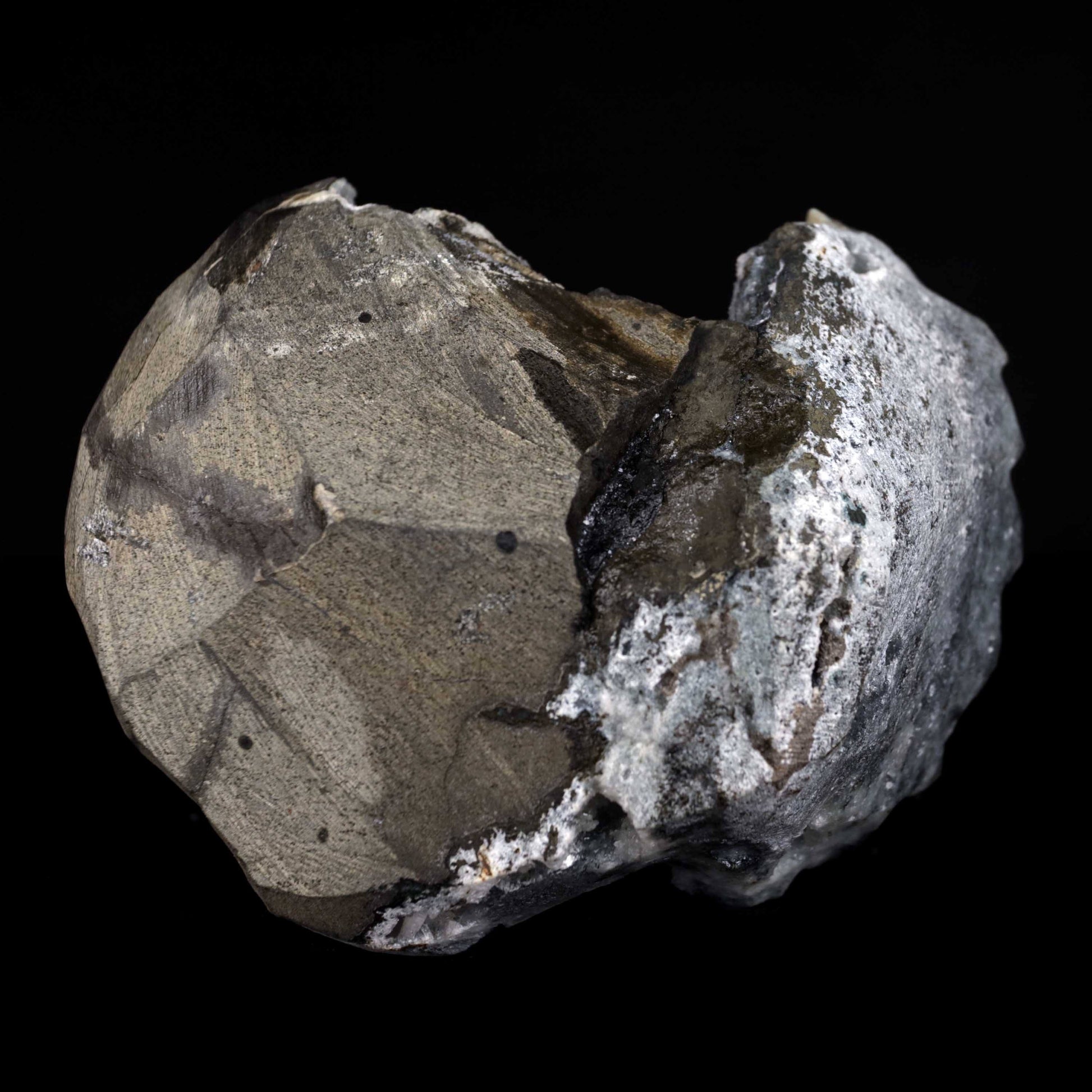This high-definition photograph captures a partial view of the interior of a rock or meteorite, likely resembling a geode. The exterior is a rough and bumpy whitish-gray with specks of brown and charred dark areas, showcasing an uneven, egg-like shape that resembles a heart. This rock is split down the middle, revealing a smooth inner texture akin to worn metal. The central chasm divides the rock into two distinct sections, the right side appearing charred gray and the left side predominantly gray. The dark, cavernous middle casts deep shadows from the lighting, enhancing the contrast against the pitch-black background, which makes the intricate and jagged edges of the exterior and the smooth interior surface vividly stand out.